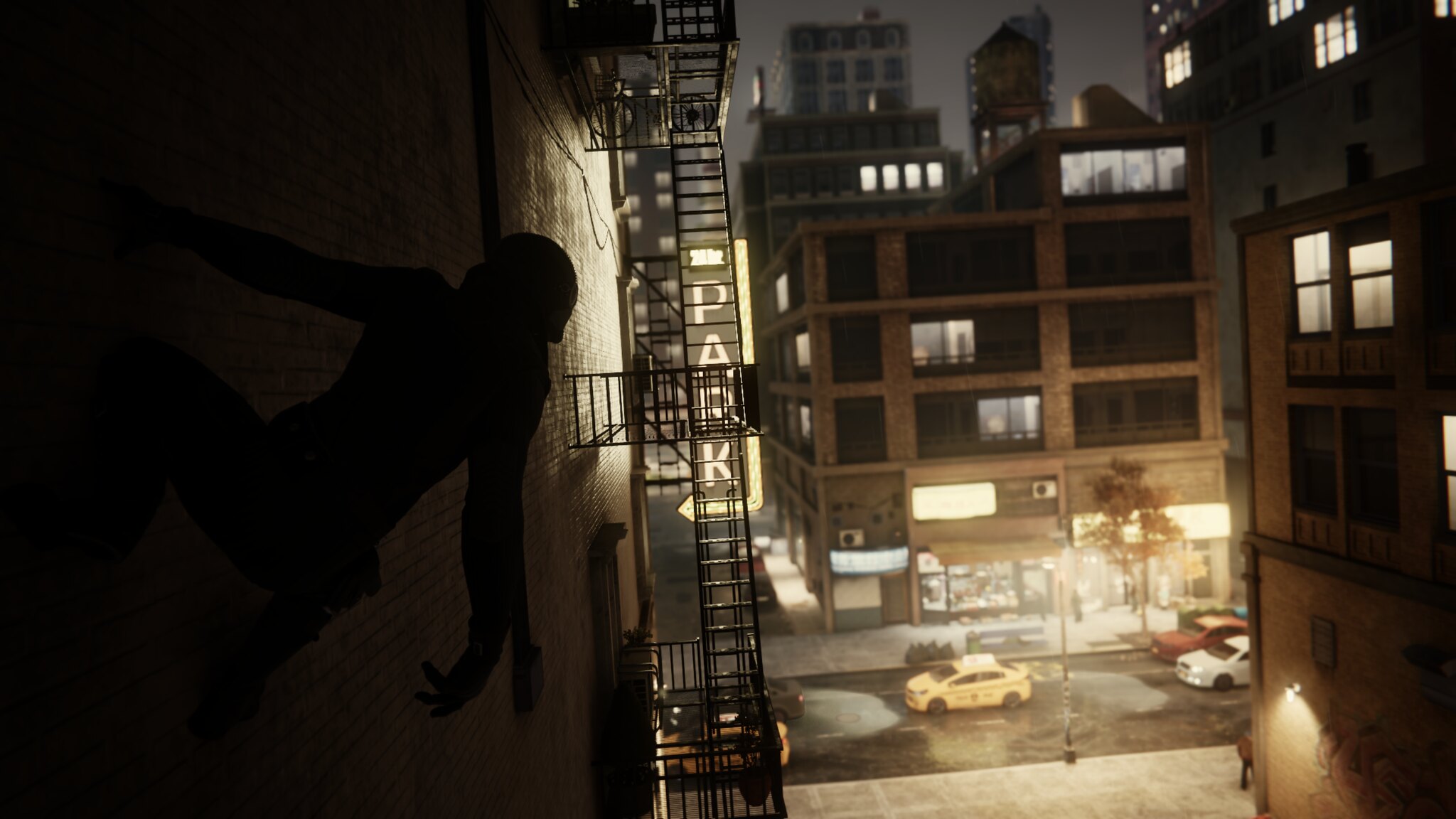In the image, a person is scaling a brick wall in a city street, seemingly without any climbing equipment. They are bald and dressed in an indistinct outfit, giving the illusion of Spider-Man-like abilities. The individual is about halfway up the wall, peering curiously over a nearby fire escape. Below on the street, various vehicles are visible, including two taxis, a red car, a white car, and a gray vehicle. Adjacent apartment buildings have their lights on, as do the skyscrapers in the background, adding an urban ambiance to the scene.